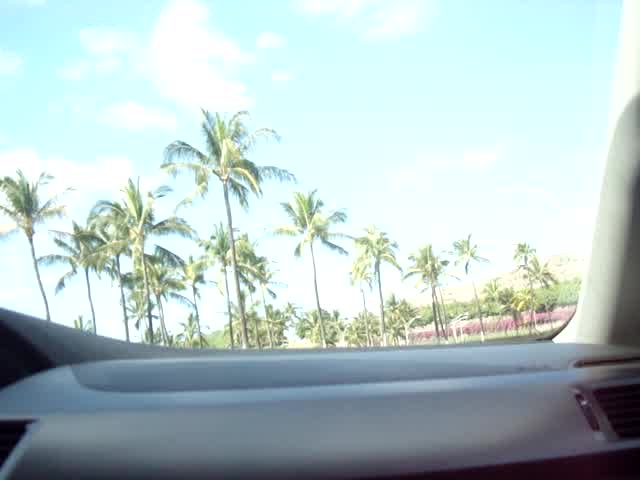The image depicts a first-person point-of-view scene from a car, likely taken from the passenger seat. The viewer's perspective includes the car's windshield, which shows a noticeable glare from the sun. The car's dashboard and heater vents, identifiable by their small control knobs, are visible on either side of the windshield. Through the windshield, the scene outside unfolds with a bright, mostly clear sky; the top right is particularly bright due to the sun. A line of tall, slender palm trees dominates the foreground, possibly around eight, with additional palm trees scattered in the background. In the scene's right-hand side, there appears to be a pink structure, either a wall or bricks, topped with grass. The overall layout and details suggest the image is being viewed through a monitor or display, possibly as part of a cartoon or hand-drawn picture.